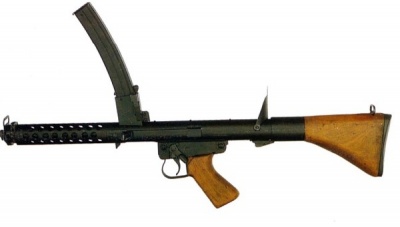The image showcases a vintage-style rifle, prominently placed against a stark white background, possibly indicative of a catalog illustration. The gun features a distinctive combination of polished wood and black metal components. The stock and handle are crafted from polished dark brown wood, offering a striking contrast to the primarily black barrel and trigger mechanism. Notably, the upper section of the gun includes a unique top-mounted magazine resembling a 'banana clip,' which is unconventional in its placement. Additionally, the rifle is equipped with a black sight near the barrel. The weapon, admired for its well-maintained condition, is positioned pointing to the left, highlighting the meticulous blend of classic design and robust utility.